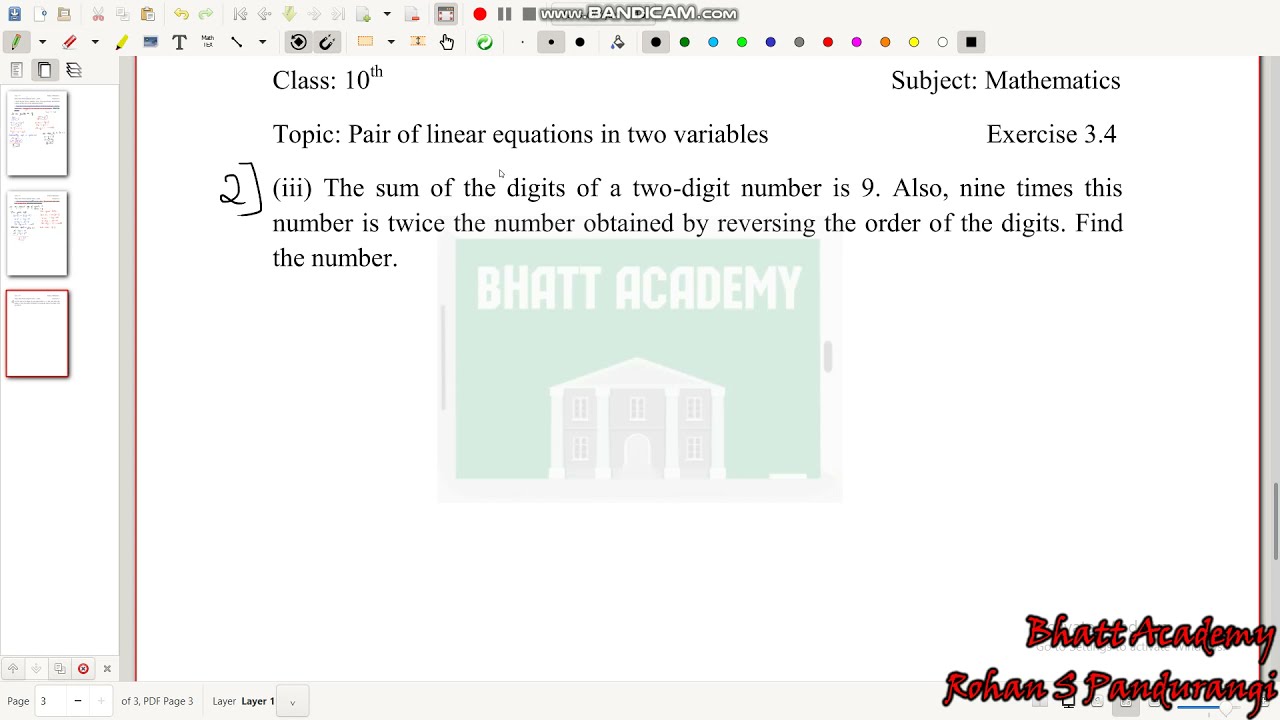The image is a detailed screenshot of a PowerPoint presentation displayed on a computer monitor. At the top center, there's a watermark with the URL "www.bandicam.com". The PowerPoint interface is visible with various icons, including a save button, print button, and a pencil.

On the left panel, there are three thumbnail pages of the presentation. The main slide in the center features the following details in black text on a white background: 

- At the top left, it says "Class: 10th".
- To the top right, it reads "Subject: Mathematics".
- Below, the text states "Topic: Pair of Linear Equations in Two Variables".
- Further down, it mentions "Exercise 3.4".
- Underneath, there's a problem description: 
  "(iii) The sum of the digits of a two-digit number is nine. Also, nine times this number is twice the number obtained by reversing the order of the digits. Find the number."

At the bottom center of the slide is a green, square-shaped logo of "BHATT Academy", featuring a house icon and text reading "BHATT Academy". Additionally, in the bottom right corner, there is red text that states "Bhatt Academy Rohan S Pandurangi", added through an editing tool.